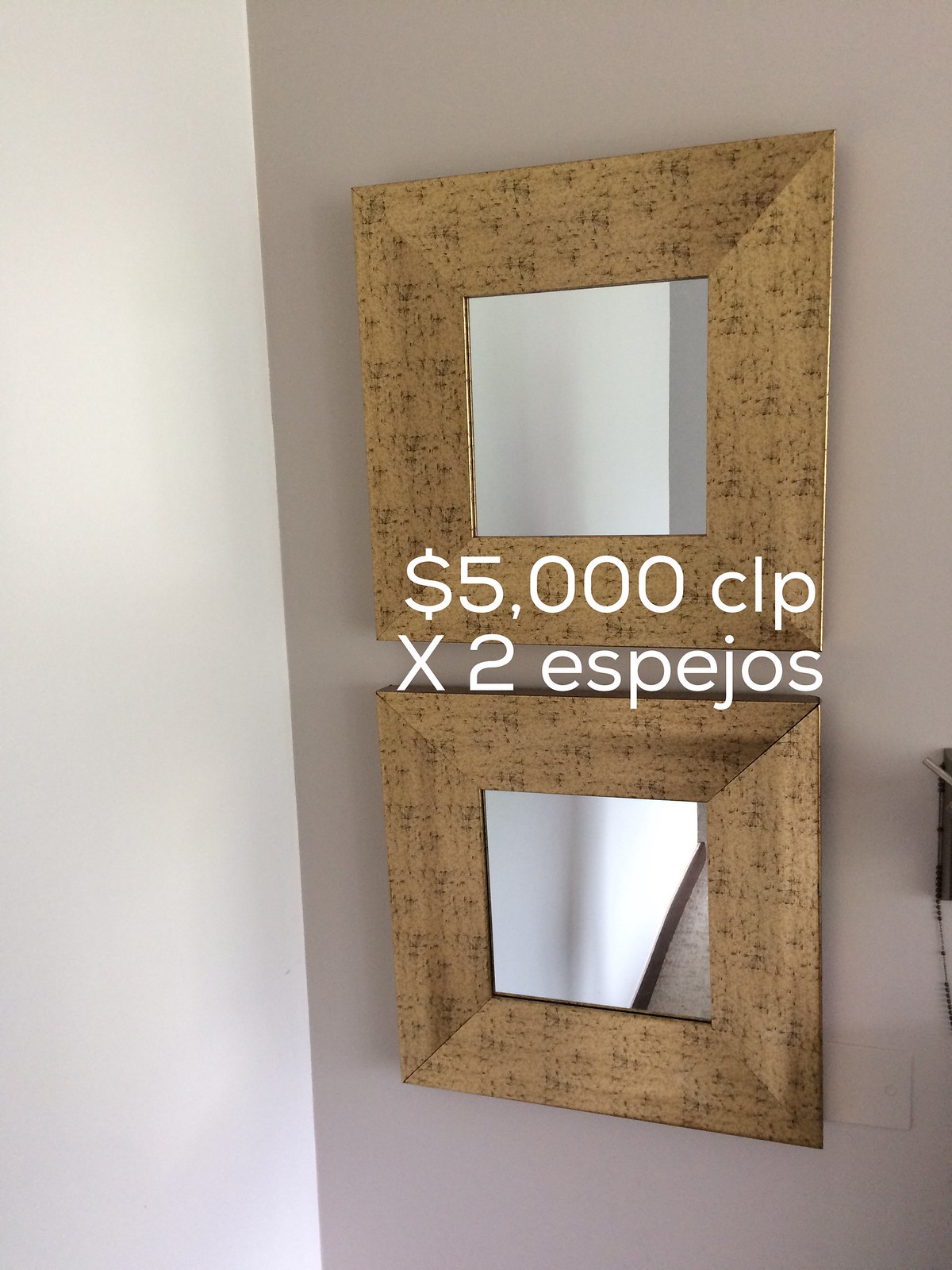The photograph features two square mirrors with a luxurious gold matte finish frame adorned with intricate black designs. These mirrors are mounted one above the other on a wall that transitions from a tan or white to a purple hue. The upper mirror reflects the adjacent wall, while the bottom mirror captures both the wall and the gray flooring below. Positioned between the two mirrors is white lettering that reads "5000 CLP x2 Espejos," indicating their price and perhaps emphasizing their high-end nature. To the right of the mirrors, partially cropped out, is a small white box and the beginning of a towel rack, partially visible but adding context to their placement. The overall color palette of the image is dominated by the gold-tan and black of the mirrors' frames, the white of the letters, and the purple and tan tones of the walls.